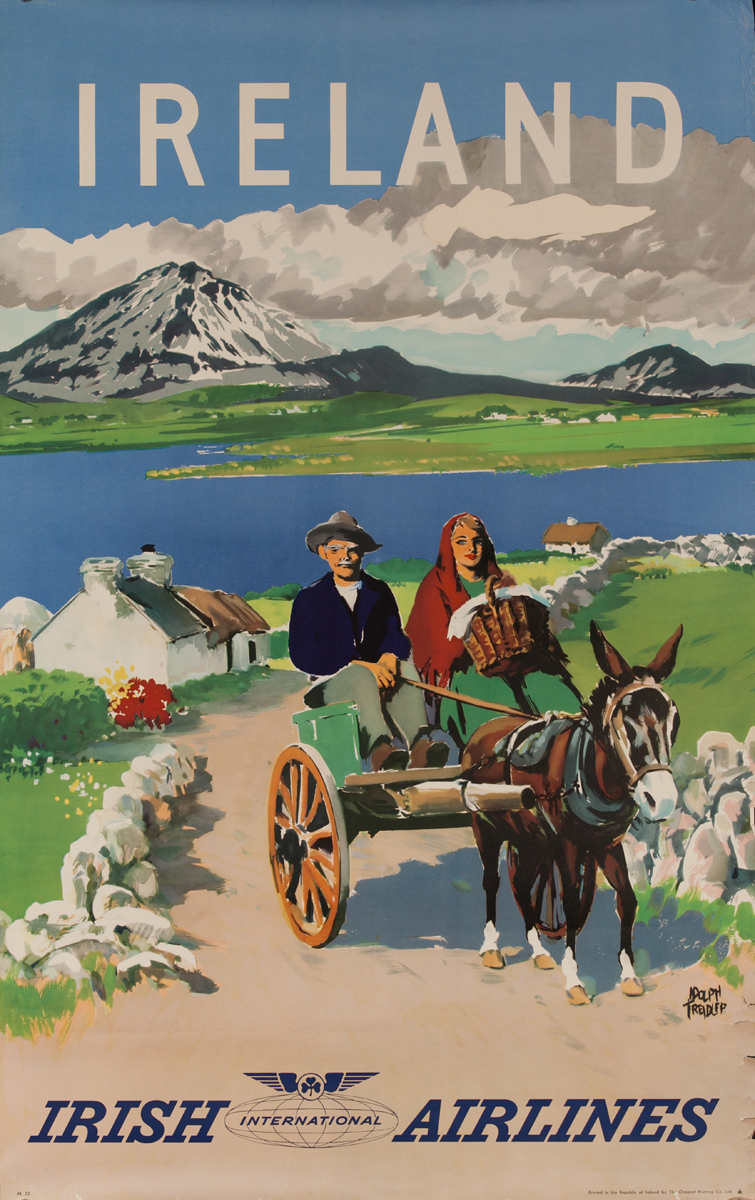This vibrant poster, reminiscent of an old-fashioned painting and classic Irish imagery, advertises Irish Airlines. At the top, the word "IRELAND" is boldly displayed in white capital letters against a bright blue sky filled with clouds. Dominating the background is a picturesque mountain range, with varying shades of gray, snow-capped peaks, and a serene river that meets a vast blue lake. In front of the mountains, there is a charming countryside scene featuring quaint cottages. Some houses have distinct roofs, with one brown, one blue, and another black; they are surrounded by green grasses, bushes, and patches of bright red and yellow flowers.

Towards the center, a rustic path winds through this idyllic setting, lined with rocks on either side. The path leads up to the viewer, where a brown donkey with a white nose and legs, outfitted with a black harness, pulls a green two-wheeled cart. Seated in the cart are two figures: an elderly man, wearing a gray hat, blue coat, white undershirt, gray pants, and brown shoes, and a woman in a green dress with a red shawl over her head and shoulders, holding a basket. The cart's wheels have brown outer rims with black centers and white sides.

At the bottom of the image, the words "Irish Airlines" are printed in dark blue font, flanked by an international logo featuring a blue clover with wings, symbolizing global connectivity. The signature "Papa dead lip" appears subtly in black on the right side of the pathway, adding a personalized touch to this nostalgic and evocative advertisement.